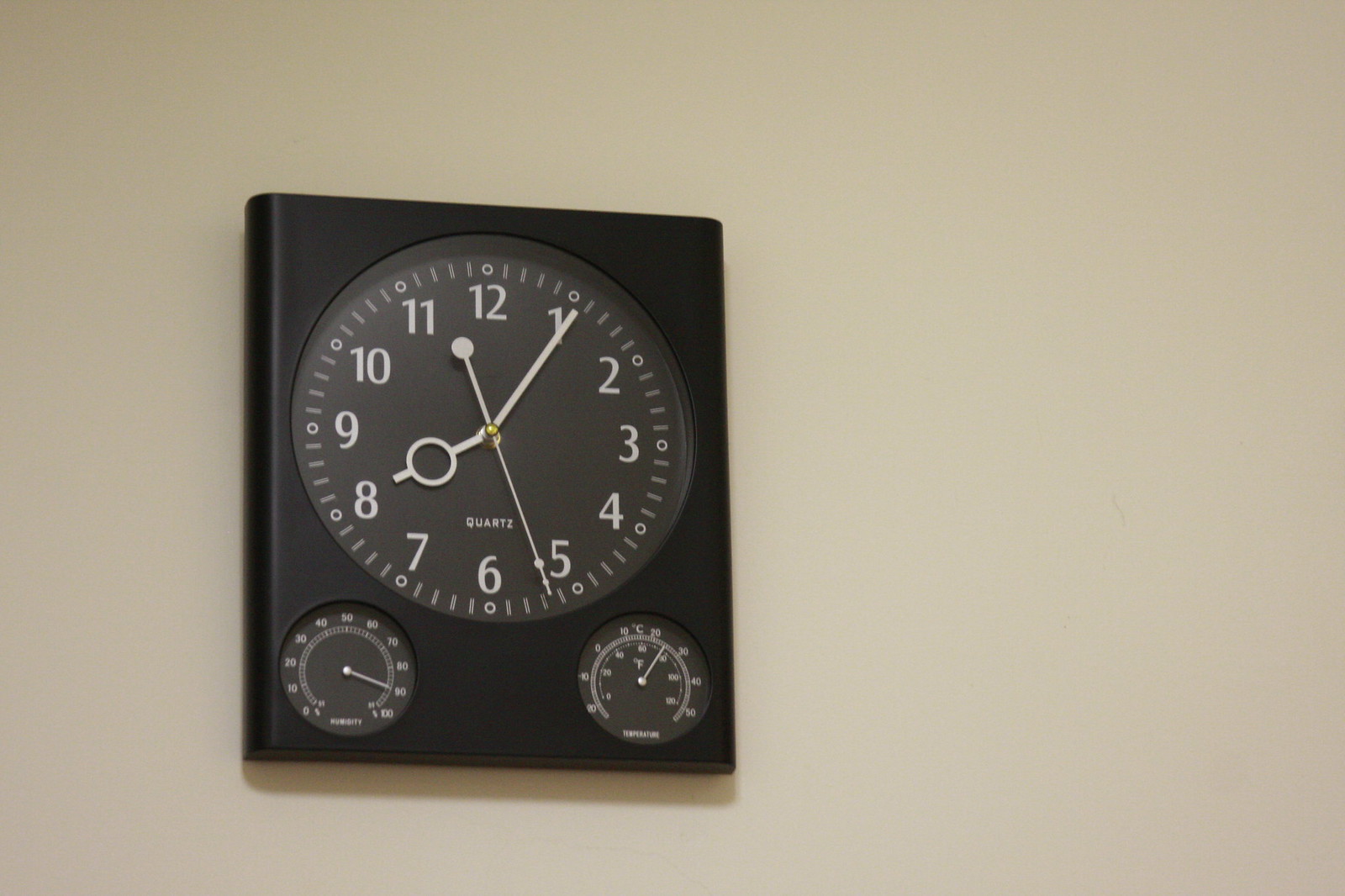The photograph showcases a black rectangular clock hanging on a cream-colored wall, positioned towards the left center of the image. The main feature of the clock is a large central round face with bold white numerals ranging from 1 to 12, and minute markers represented by lines. The current time displayed is 1:26. The hour hand has an interesting design, resembling a stick figure with an 'O' in the middle, and both the hour and minute hands are simple white lines. The second hand is distinguished by small circles at each end. Beneath the main clock face, the word "quartz" is inscribed. Additionally, there are two smaller round dials at the lower part of the clock: one on the left indicating humidity levels from 0 to 100, and one on the right showing temperature in Celsius.